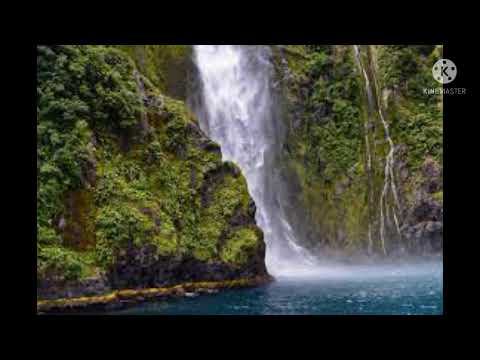The photograph features a breathtaking tropical waterfall cascading down into a serene, dark blue lagoon. The waterfall, which dominates the center of the image, is abruptly cut off at the top, leaving its source unseen. The water rushes down rapidly, manifesting as a powerful stream of white water that creates a misty haze where it meets the lagoon's surface. On either side of the waterfall, the cliffs are covered in lush, verdant vegetation, contributing to the tropical ambiance.

To the left of the waterfall, a prominent rock formation juts out, partially obstructing the base of the cascade. This rock is blanketed in green moss or grass, enhancing its natural beauty. On the right side, additional rock formations rise vertically, adorned with more greenery and possibly a vine-like growth clinging to the cliff. The overall backdrop is filled with dense vegetation, illustrating a thriving and vibrant ecosystem.

The image is framed by a solid black border, adding a distinctive touch. Additionally, a watermark featuring a white circle and some illegible text, possibly resembling a clock with two hands, is visible in the upper right corner, extending slightly into the photograph. The bright midday sun illuminates the entire scene, casting a beautiful, natural light over the water and vegetation, further emphasizing the vivid colors and dynamic movement within the image.